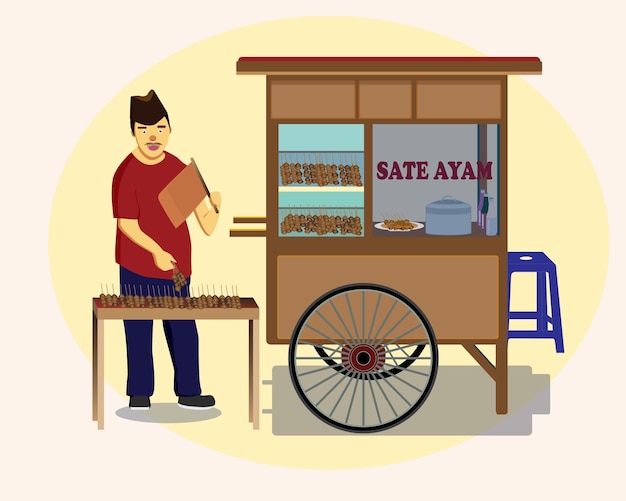This is a detailed, computer-generated, cartoonish image of a street vendor standing next to his food cart. The background is a soft pink shade, with a pale peach-yellow circle highlighting the central elements. To the left stands a man, possibly of Chinese descent, dressed in a black cap, a red shirt, navy blue pants, and black sneakers with white soles. He holds a small, brown flag in his left hand. 

The vendor is positioned behind a brown table displaying around 20 to 30 skewers of meat, possibly beef jerky or bacon skewers. Adjacent to him on his left is a brown cart with two black wheels, featuring two layers of skewered meat inside. The cart has the words "satay ayam" (Indonesian for chicken satay) written on its side. Next to the cart, on its right, is a royal blue-colored stool. The overall image is simplistic and cartoon-like, portraying the vibrant essence of a street food scene.